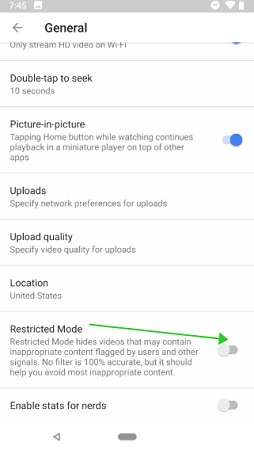The image is a screenshot of a mobile device displaying various video settings options. At the top of the screen is a thin gray bar indicating the time as 7:45. Below this bar, a white strip features the word "General" in black text, accompanied by a left-facing arrow on the far left.

The settings are organized into sections, each separated by thin horizontal gray bars:

1. **Stream HD Video Only on Wi-Fi:**
   - Indicates an option related to streaming high-definition video exclusively over Wi-Fi connections.

2. **Double Tap to Seek:**
   - Specifies a feature that allows users to skip ahead by 10 seconds with a double-tap gesture.

3. **Picture-in-Picture:**
   - Describes a functionality where tapping the home button while watching a video will continue playback in a miniature player overlay, usable alongside other apps.
   - Includes a blue slider to enable or disable this feature.

4. **Upload - Specify Network Preferences for Uploads:**
   - Refers to settings where users can determine network conditions for uploading videos.

5. **Upload Quality:**
   - Allows specification of video quality for uploads.

6. **Location:**
   - Indicates the current set location, which is the United States.

7. **Restricted Mode:**
   - Provides details about a mode that hides videos potentially containing inappropriate content flagged by users and other signals.
   - States that it isn't 100% effective but should help avoid most inappropriate content.
   - Features a gray slider with a green arrow pointing to it.

8. **Enable Stats for Nerds:**
   - Describes an option to display detailed video statistics.
   - Comes with a gray slider to toggle the feature.

At the bottom, there is a small gray bit, which is likely a portion of the interface or additional settings.